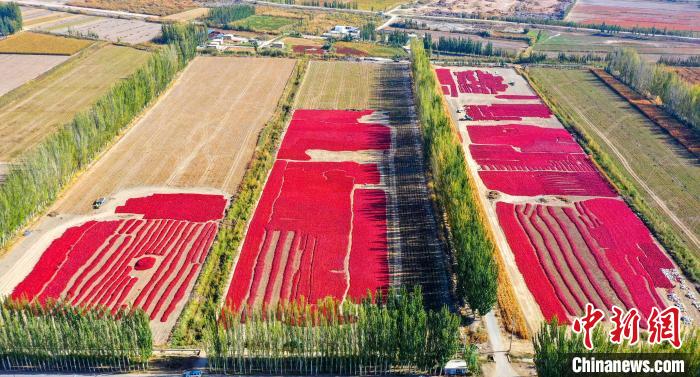This aerial photograph, likely taken from a drone or plane, captures a sprawling agricultural landscape. The central focus is a series of rectangular fields, segmented by tall, pencil-shaped trees. Among these fields, three main plots stand out prominently: the first features red plants occupying the lower third, the second has red plants covering about two-thirds, and the third is almost entirely blanketed in these vibrant red plants. Rows of white soil or pathways separate these vividly colored sections. The surrounding areas are predominantly green, possibly indicating different crops or vegetation. In the distance, a few scattered buildings can be seen amidst more green vegetation. Shadows cast by the sun enhance the natural texture of the scene. Overlaying the image, there is text in both Chinese and English, with "Chinanews.com" clearly visible at the bottom right, signifying the source of the photograph.